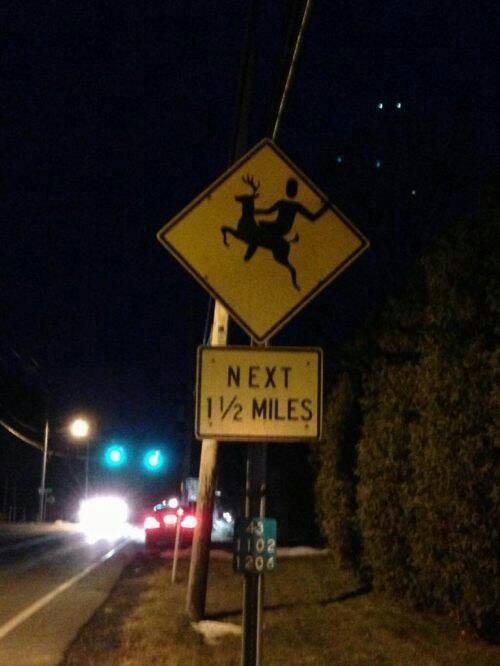The image depicts a detailed roadside scene. On the right side of a two-lane road, a quirky street sign captures attention. The sign, positioned just in front of a power pole, features a diamond-shaped, yellow caution sign with a humorous illustration of a person riding a bucking reindeer, resembling a rodeo act. Beneath it, a rectangular sign reads "Next 4.5 miles." The road itself stretches into the distance with a traffic light visible approximately fifty yards ahead. Near the sign, a car is pulled over onto an unpaved shoulder, its brake lights glowing red. The surrounding landscape includes thin grass, possibly with some snow patches, indicating an off-season, and a few scattered shrubs to the right. In the distance, on the left side of the road, a street light is faintly visible.